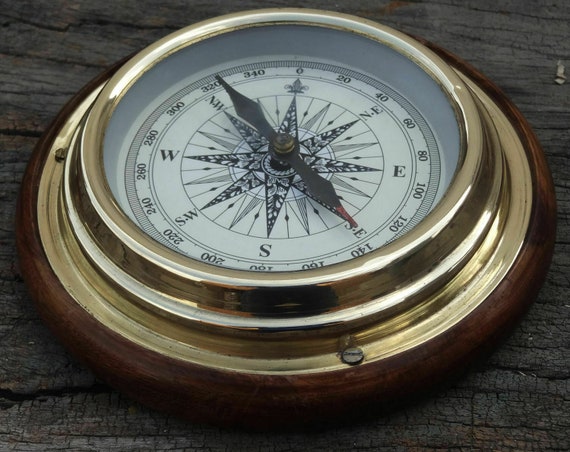This image captures a detailed close-up of an elegant brass compass, showcasing both its intricate design and functionality. The compass, crafted from a blend of brass and wood, features a round, polished brass casing juxtaposed with the natural texture of wood. The compass interface, protected by a clear glass cover, displays a classic navigational layout characterized by a striking black and white motif.

The needle of the compass is meticulously designed, with one end pointing to the Southeast (SE) direction, marked by a small red tip, while the opposite end points towards the 320-degree mark, colored entirely in black. The interface is adorned with a star-shaped central design in contrasting black and white, enhancing its aesthetic appeal.

The numerical markers on the compass range from 0 to 340 degrees, providing precise measurement capabilities. Additionally, the compass indicates cardinal directions—Northeast (NE), Southeast (SE), Southwest (SW), Northwest (NW), West (W), East (E), South (S), offering a complete and accurate reading for navigation. This sophisticated device exemplifies both traditional craftsmanship and practical use, making it a timeless tool for explorers and navigators alike.